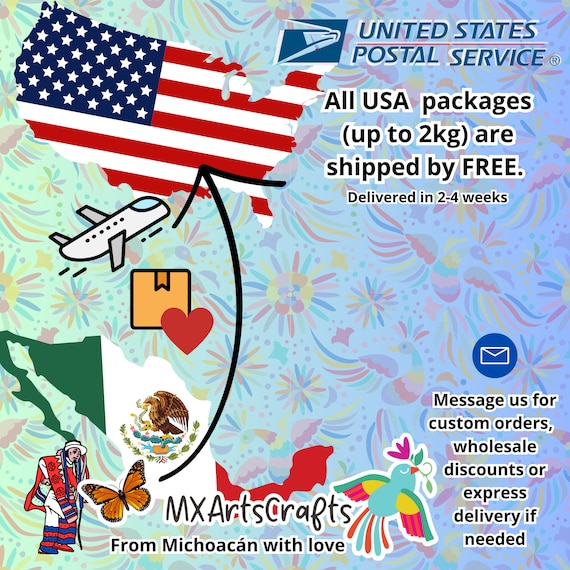This vibrant advertisement for the United States Postal Service prominently features a colorful, watercolor-like background reminiscent of fireworks and streamers. On the top left, there's sizable clipart of the United States, patterned like the American flag, beside the USPS logo. The text next to the logo announces that all USA packages up to 2 kilograms are shipped for free, with delivery times ranging from 2 to 4 weeks. The bottom right corner showcases the MX Arts Crafts logo, stating "From Michoacan with Love." An envelope is also depicted here, accompanied by an invitation to message for custom orders, wholesale discounts, or express delivery options. The poster features additional cartoon-style elements: a heart, an airplane traveling from a map of Mexico—illustrated in the nation's green, white, and red colors with an eagle clutching a snake—towards the U.S. Between these maps is an arrow symbolizing the delivery route. Completing the scene, a man dressed in traditional Mexican attire appears, emphasizing the cultural connection between the artisans of Michoacan and their U.S.-based customers.